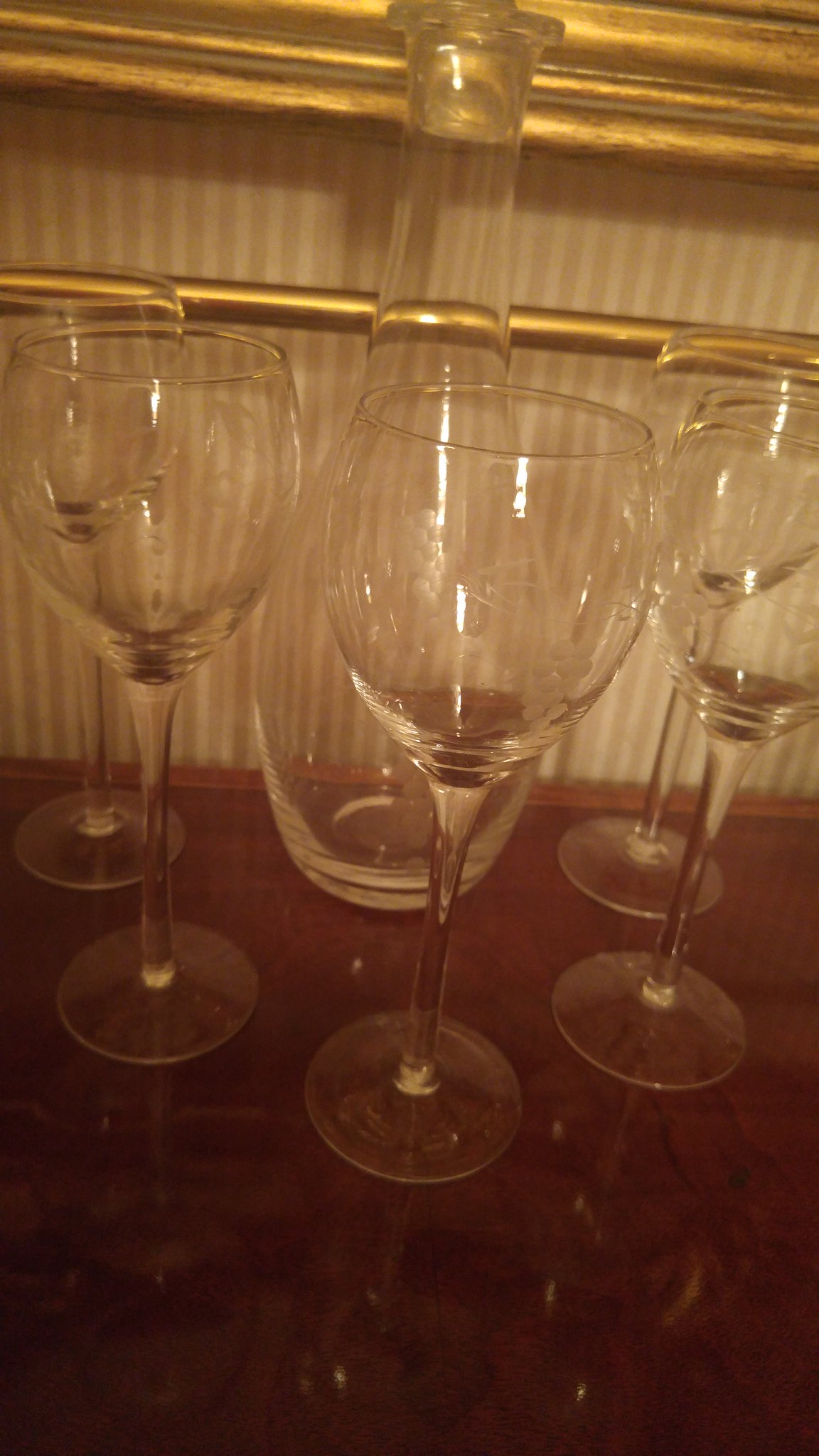This photograph, slightly skewed to the right, captures a meticulous arrangement of glassware on a shiny brown wood-look tabletop. At the center, a glass carafe with its top slightly cut off is flanked by five identical clear wine glasses forming a semi-circle. The setting is framed by a wall featuring vertical cream and light brown pinstripes, accented by a gold leaf chair railing and a matching gold leaf picture frame just visible at the top of the image. The scene appears clean and organized, suggesting a deliberate setup rather than the aftermath of a wine-drinking session. There's no text in the image; the focus is solely on the elegant display of glassware.